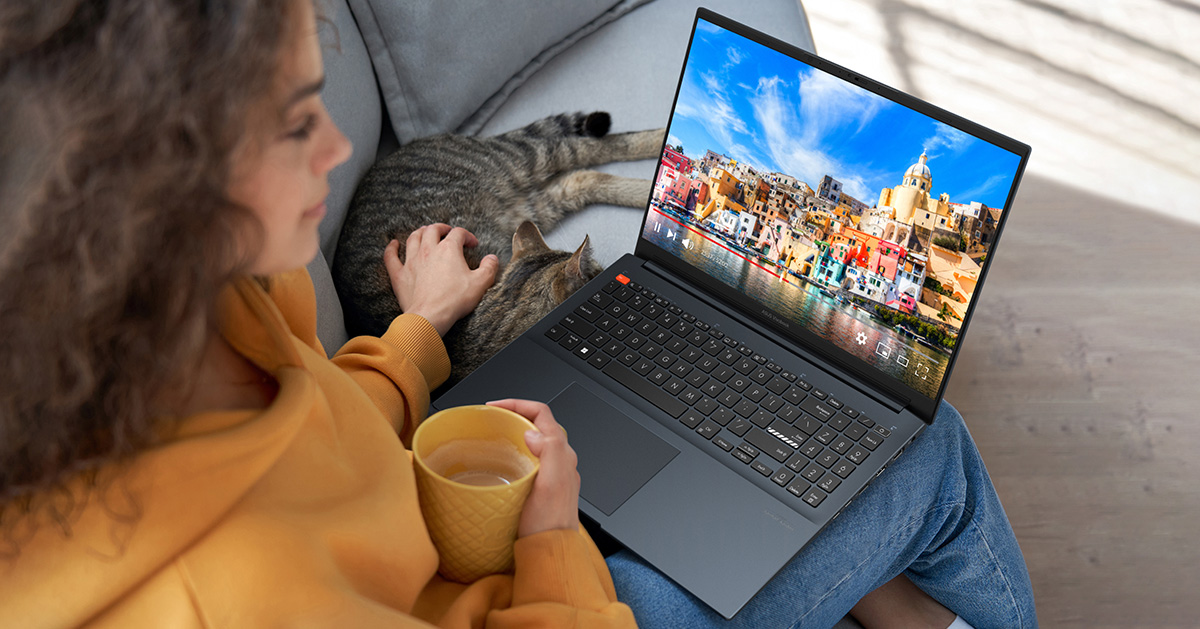In the photograph, a woman with long brown hair sits on a chair, facing slightly to the right. She is wearing a yellow-orange hoodie and holding a yellow-orange mug in her right hand, which appears to contain coffee with a lot of creamer. Her left hand gently pets a dark gray cat with black stripes that is sitting beside her on the couch. Resting on her lap is a mostly black laptop. The laptop screen displays an image of a dense, compact city with buildings of various colors, situated by a body of water. The sky in the image is a vibrant blue with a few wispy white clouds. Sunlight illuminates the floor, suggesting that the photo was taken during the day, possibly outside or in a well-lit room. The image is taken from an angle above her shoulder, providing a detailed overhead view of her and the laptop screen.